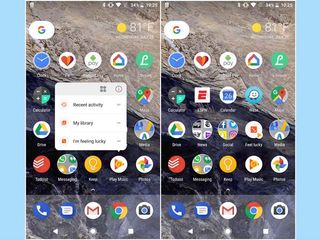The image features two side-by-side screenshots of an identical smartphone home screen or app drawer. The screenshot on the left displays the Google Play Music app icon being highlighted or long-pressed, which activates a context menu. This menu presents several options: a circular "i" button for information, "Reset Activity," "My Library," and "I'm Feeling Lucky." Conversely, the screenshot on the right shows the same home screen layout but without the context menu displayed. Both screenshots capture the identical phone setup with the same background, apps, and icons, emphasizing the specific interaction with the Play Music app in the left screenshot.